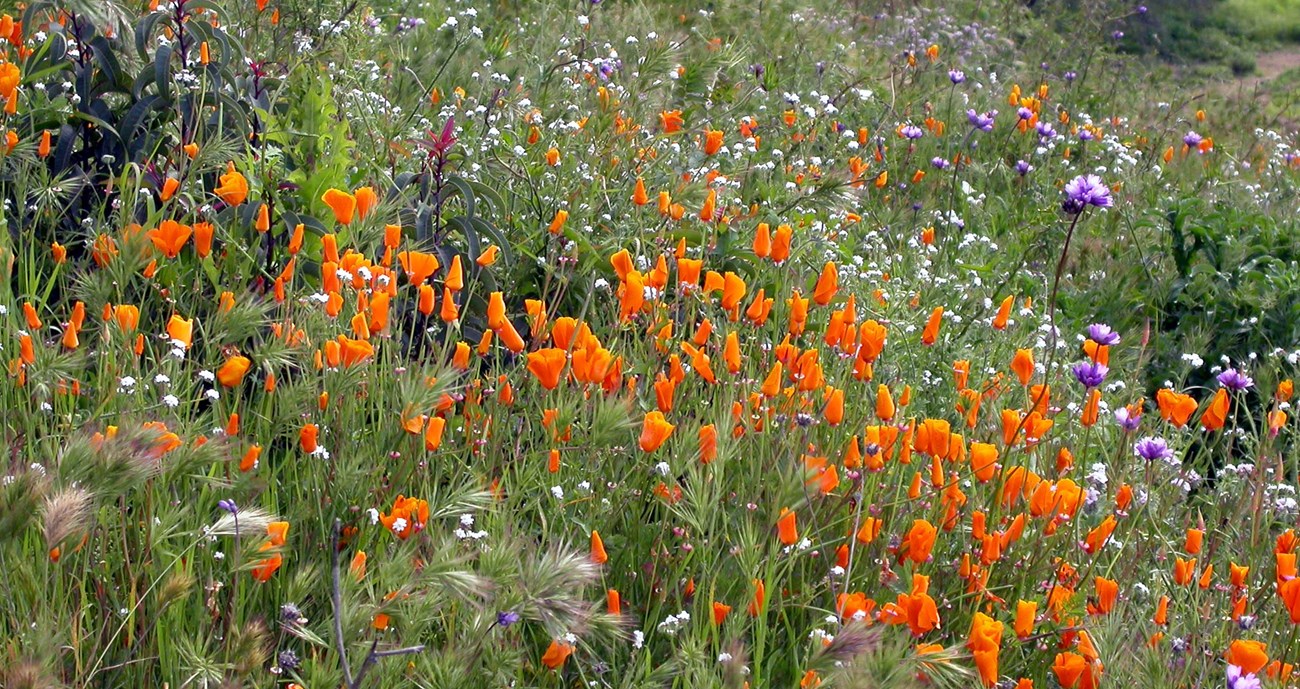This vibrant photograph depicts a colorful meadow abundant with various types of wildflowers. Dominating the scene are radiant orange tulips, stretching from the top left to the bottom right, surrounded by a lush array of greenery. Scattered among the tulips, there are delicate purple flowers with small petals and clusters of white flowers in the background. Near the top left, a dark-leaved plant with banana-shaped leaves provides a stark contrast to the bright floral colors, while at the center, a plant with reddish leaves adds another layer of visual interest. Additional plants resembling tall rushes add texture to the scene. In the upper right corner, a small dirt path slightly peeks through the lush foliage, hinting at a serene walkway, with the vibrant meadow serving as a natural retreat for visitors to enjoy. The intricate details and variety of the flora create a striking and harmonious display of nature’s beauty.